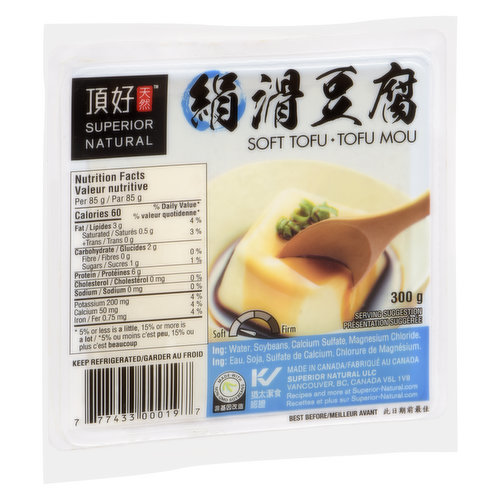This image showcases the packaging of a soft tofu product, prominently displayed in a clean and detailed manner. The packaging features bilingual text (English and French), with the brand "Superior Natural" highlighted at the top left, accompanied by a black box with non-English text likely in Japanese or Chinese. Below this, "soft tofu" is clearly stated. The package also depicts a photograph of a serving suggestion: a blob of tofu in a bowl, topped with a sauce, into which a brown spoon is inserted. 

Nutritional information is meticulously detailed in the Nutrition Facts box on the left, listing 60 calories, 3 grams of fats (including 0.5 grams of saturated fat), 2 grams of carbohydrates, and 6 grams of protein, with no cholesterol or sodium. The mineral content includes 200 mg of potassium, 50 mg of calcium, and 0.75 mg of iron. The packaging also emphasizes that the total serving size is 300 grams.

The lower left corner of the package features a barcode and a note to keep the product refrigerated. Below the photograph, the ingredients—water, soybeans, calcium sulfate, and magnesium chloride—are listed, repeated in French as well. The product is manufactured by Superior Natural Corporation located in Vancouver, British Columbia, Canada.